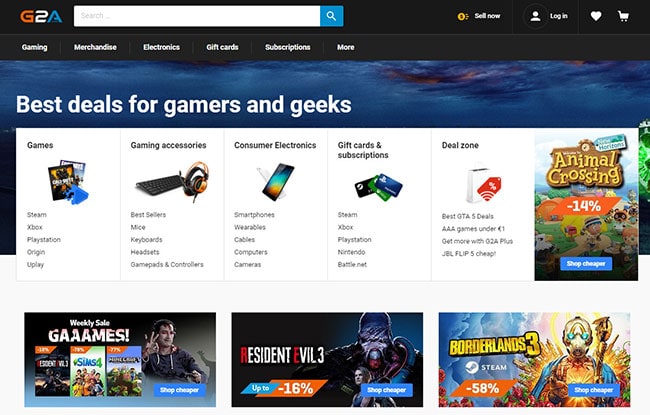Screenshot of the G2A Website:

The image depicts a screenshot of the G2A website, a popular platform for gaming products. Dominating the upper part of the page, a sleek black header is accompanied by a dark gray menu bar right below. At the very top is a white search bar featuring a blue magnifying glass icon for initiating searches. Adjacent to the search field are icons for various functionalities, including "Sell Now," "Login," a "Heart" for likes, and a "Shopping Cart."

The menu bar provides comprehensive navigation options, including categories such as Gaming, Merchandise, Electronics, Gift Cards, Subscriptions, and more. Just below the menu, a vibrant banner image depicting reflective water proudly announces, "Best deals for gamers and geeks."

An overlay panel is superimposed on the banner, showcasing several prominent categories: Gaming, Gaming Accessories, Computer Electronics, Gift Cards & Subscriptions, and Deal Zones. Under the Gaming section, various boxed thumbnails represent platforms like Steam, Xbox, PlayStation, Origin, and Uplay. Gaming Accessories feature visual representations of a keyboard and headsets, while Consumer Electronics display images of phones and tablets. Gift Cards are symbolized by credit card icons, and Deal Zones are marked by sales tags.

Highlighting some specific offers, the right side of the image advertises "Animal Crossing" at 14% off. Further down the page, three graphic thumbnails promote weekly sales and featured deals. These include an array of games such as "The Sims," "Resident Evil," and another unspecified game with a character making an OK gesture. The middle thumbnail highlights "Resident Evil 3" with discounts up to 16% off, and the rightmost thumbnail showcases "Borderlands 3" on Steam, available at 58% off, urging viewers to "Shop Cheaper."

The visually rich layout and detailed navigation options make it clear that G2A is dedicated to providing a wide range of deals for gaming enthusiasts.